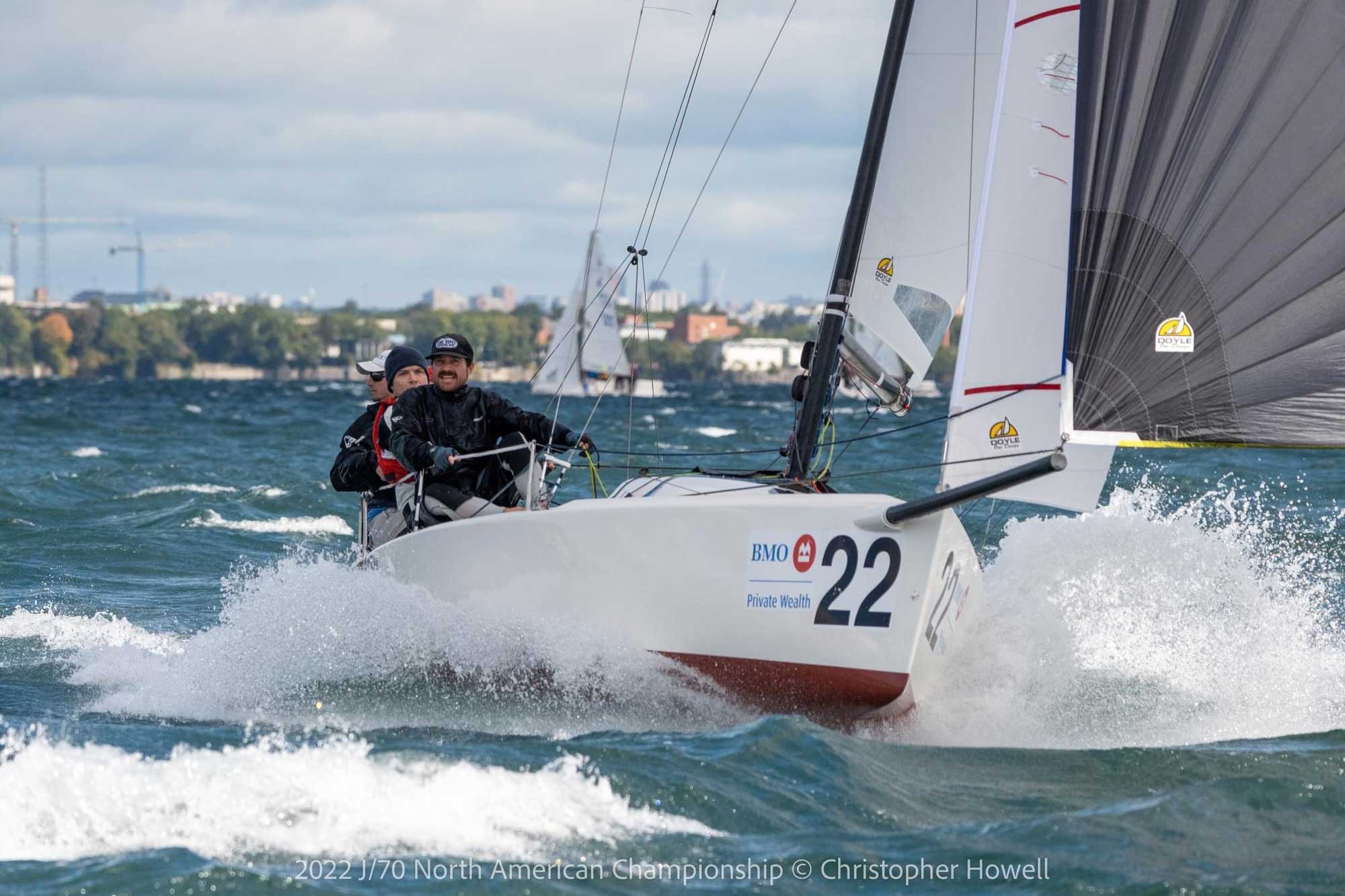This is a detailed color photograph capturing three men sailing a white sailboat. Prominently visible on the bow are the red text "BMO" with a red logo beside it, and "Private Wealth." In large black text, the number "22" is displayed, and the mast, which is black, rises in the center with visible rigging extending upwards. To the right of the mast, there's a transparent black sail and a white sail positioned behind it. To the left, leaning on a silver metal rail, are three men: the one in front wears a black jacket and a baseball cap, the second man sports a mint-colored cap, and the third has a white baseball cap. The sailboat is creating white waves as it moves through blue water dotted with whitecaps, and another sailboat can be seen in the background. Onshore, trees and buildings are visible under a cloudy sky. Further details include a mention of the sails branded with the Doyle logo, depicting a half-dome-shaped sun with sailboats, and text reading "2022 J-70 North American Championships. Copyright, Christopher Howell," displayed at the bottom left of the image.